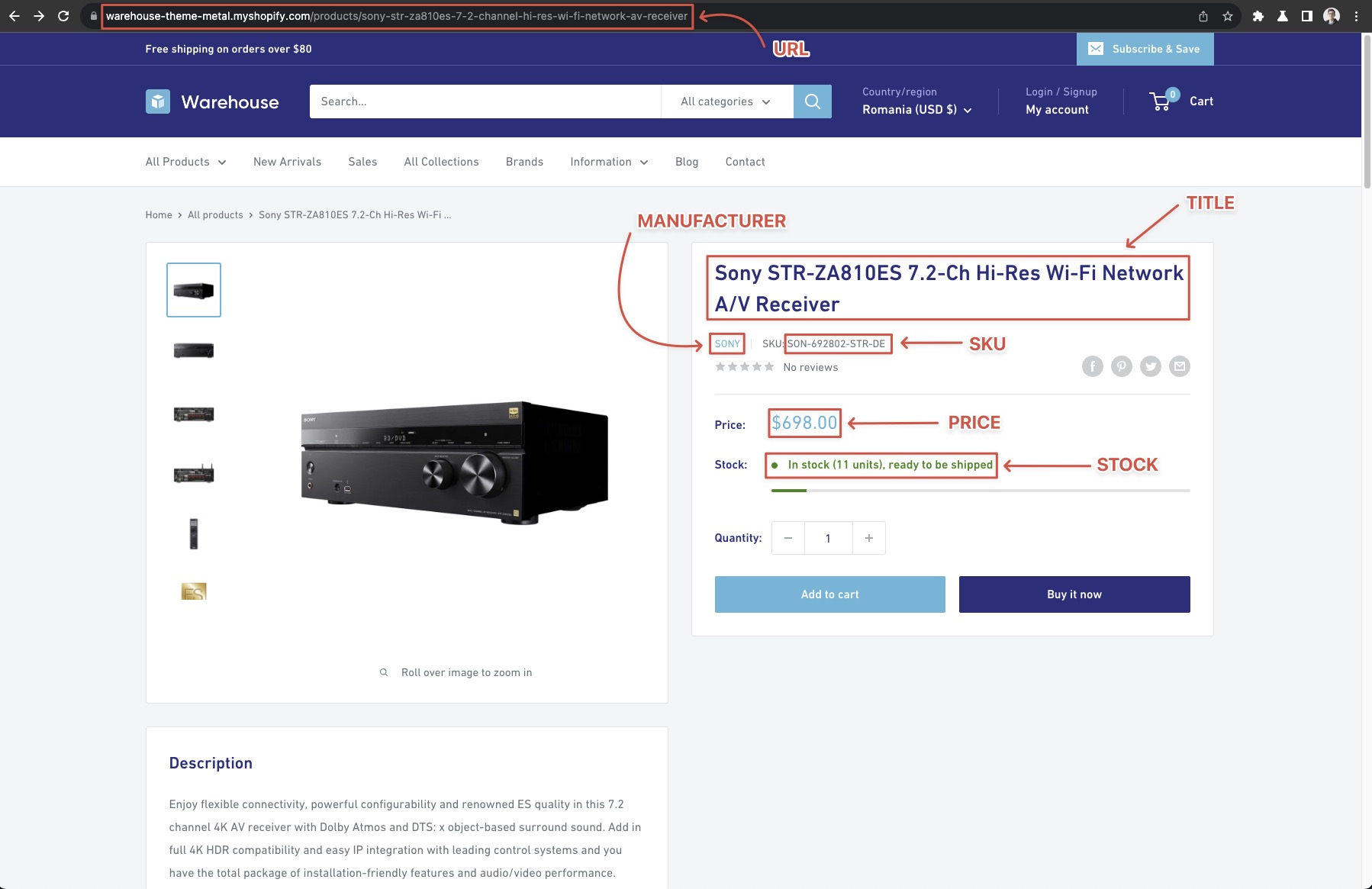**Caption:**

This screenshot captures a section of a warehouse website, featuring the 'Warehouse-Theme-Metal' template on the Shopify platform. The Shopify platform enables global product sellers to reach a diverse clientele, operating across countries. At the top of the webpage, navigation elements include a web address, a group of icons in the right corner, a username field, and icons for a puzzle, star, and a download button.

Below these elements, a light blue "Subscribe and Save" button is prominently displayed. Adjacent to this, there is a cart icon indicating zero items, alongside options for logging in and selecting the country, which may also influence the language displayed on the site.

The highlighted product on this page is a Sony AV receiver, specifically a black, heavy model designed for home theater setups. The receiver features two round knobs on the front panel, an interface screen, and a DVD slot. To the left of the main product image, additional images provide different views of the receiver. The product is identified as a Sony STR receiver, with the manufacturer indicated as Sony. Below this, specific SKU numbers are listed, and the price is marked at $6.98. The item is in stock, with 11 units ready to ship. Beneath the product description, options to "Add to Cart" and "Buy Now" are available.